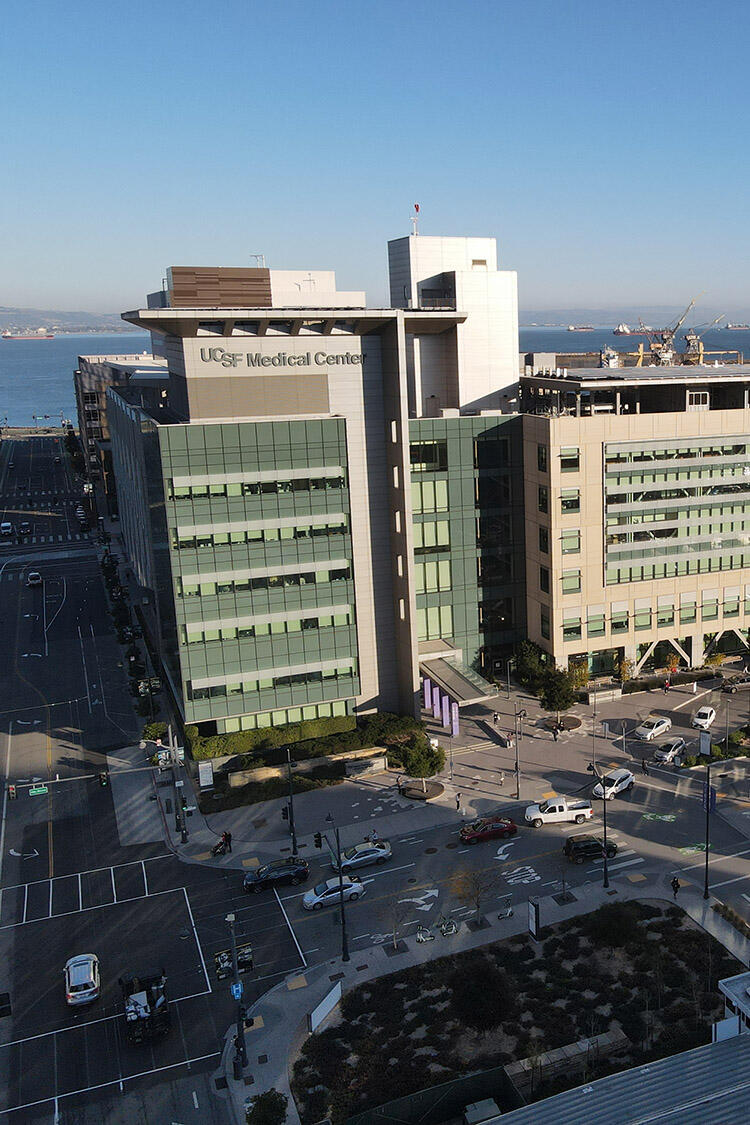The aerial photograph captures the UCSF Medical Center, a tall multi-story hospital comprised of a variety of rectangular shapes. The building prominently displays the name "UCSF Medical Center" in black letters at the top. The structure is distinctly divided into two sections: the left side is green and gray with green-tinged windows, many adorned with different states of pulled-down curtains, while the right side is beige, featuring a large gray platform seemingly designated for helicopter landings. The hospital building is set against the backdrop of the San Francisco Bay, where multiple cranes and cargo ships are visible on the blue waters. Below, the photograph shows a busy city street, complete with cars navigating through an intersection with traffic lights. On the lower left side, there is a parking lot, and on the lower right, a patch of land, possibly part of a ledge or wall. The scene is set under a clear blue sky, enhancing the vibrant details of the hospital and its surroundings.